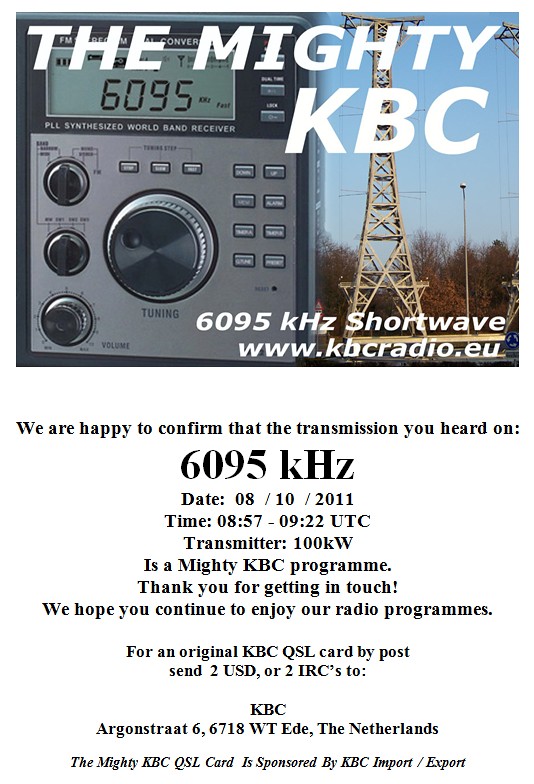The vertical rectangular advertisement for The Mighty KBC radio station features a close-up photograph of a green radio on the left-hand side, with visible tuning and volume knobs along with several buttons. The radio screen prominently displays "6095 kHz" along with indicators for network and battery status, and the label "PLL Synthesized World Band Receiver" beneath the screen. Adjacent to the radio on the right side of the photograph is an image of a large transmission tower set against a backdrop of blue sky and trees. At the top of the image, large white bold letters proclaim "The Mighty KBC." Below the photograph, the text reads "6095 kilohertz shortwave" with the website "www.kbcradio.eu" underneath. Further down, against a white background, the text confirms a broadcast at the specified frequency: "We are happy to confirm that the transmission you heard on 6095 kilohertz," followed by "Date: 08/10/2011 Time: 0857 to 0922 UTC Transmitter: 100 kilowatts is a Mighty KBC program. Thank you for getting in touch; we hope you continue to enjoy our radio programs. For an original KBC QSL card, send $2 USD or two IRCs to KBC Argenstrasse 6, 6718 WT, EDE, The Netherlands." The footnote mentions that the QSL card is sponsored by KBC Import/Export.